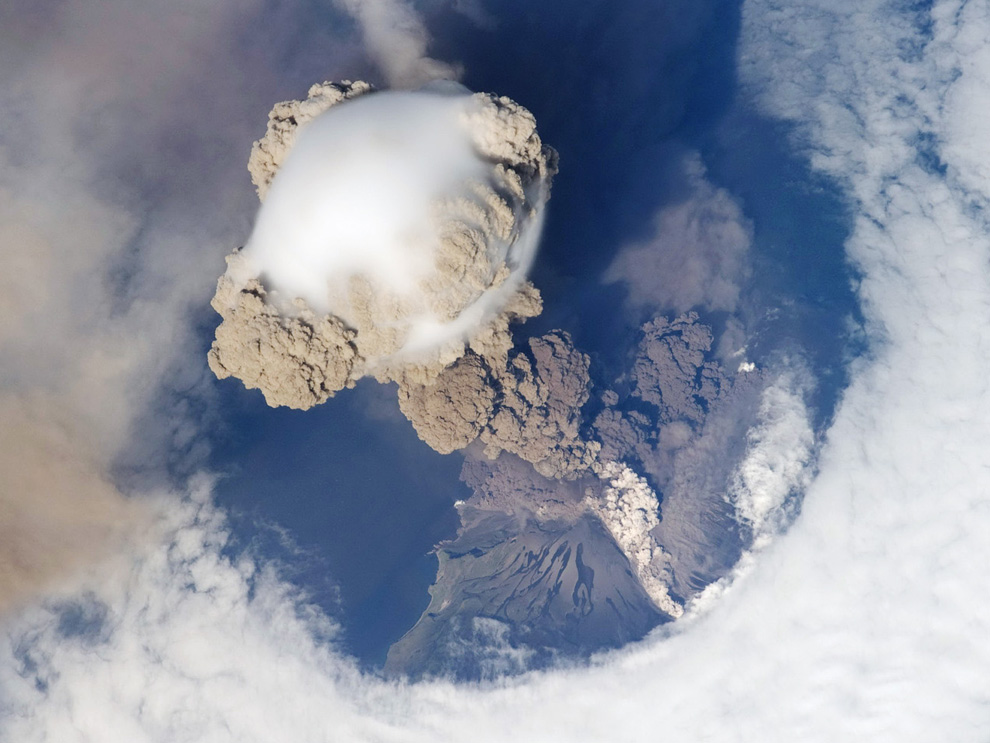This aerial photograph, taken from an altitude of approximately two to three miles, captures a dramatic volcanic eruption. A towering pillar of dark brown volcanic ash surges upwards from the ground, centered in a circular opening within a blanket of white clouds. This striking cloud formation expands outward, resembling a giant mushroom cloud with a white, smoky core surrounded by beige and brown ash. The scene on the ground, partially visible through the opalescent gap in the clouds, reveals a landscape potentially covered with green and spotted with blue haze. Additional smaller, dark gray clouds linger around the edges, further accentuating the magnitude of this explosive natural event.